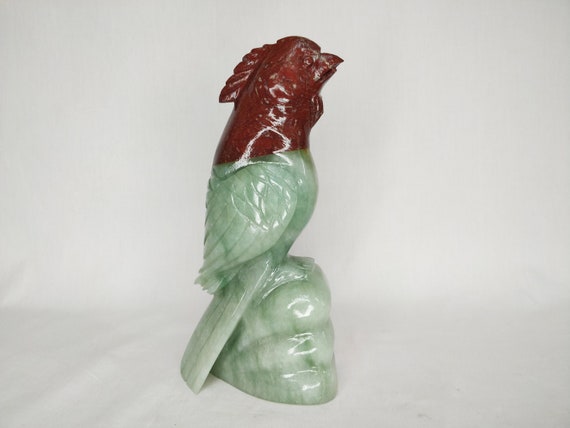This image features a vintage-style miniature statuette of a bird, possibly a chicken, perched on a rock. The figure is intricately crafted with two distinct colors—red and a light jade-like green. The bird's head, neck, and the feathers at the top are made of a red stone, while the body, wings, and tail are of the same jade-like stone as the rock it stands on. The statuette is positioned against a white cloth backdrop, suggesting it might be a product for sale, possibly on an online site or in an antique store. The detailed and contrasting materials give it a unique, collectible appeal.